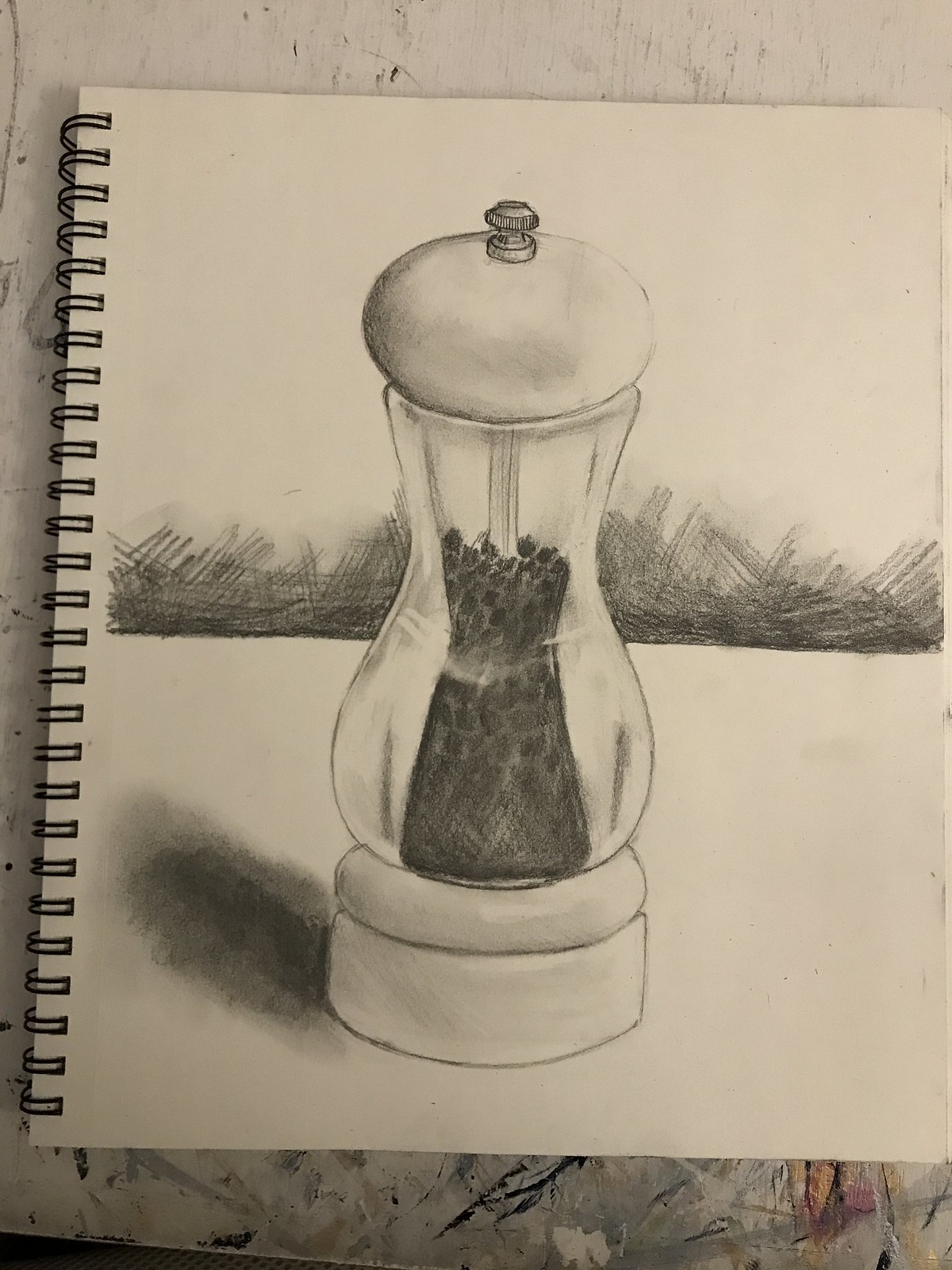A meticulously detailed pencil drawing is captured in this photograph, which showcases a piece of paper in a spiral-bound notebook resting on a table surface. The drawing features a transparent pepper grinder, allowing a clear view of the peppercorns housed within its inner chamber. The grinder stands upright on a drawn table, casting a shadow to its left, adding depth and realism to the composition. The cylindrical body of the pepper grinder reveals an intricate central stem, crucial to its grinding mechanism. Atop this structure sits a bulbous knob, crowned with a smaller metal knob protruding from its peak. The background is subtly shaded, providing contrast and enhancing the overall dimensionality of the artwork.